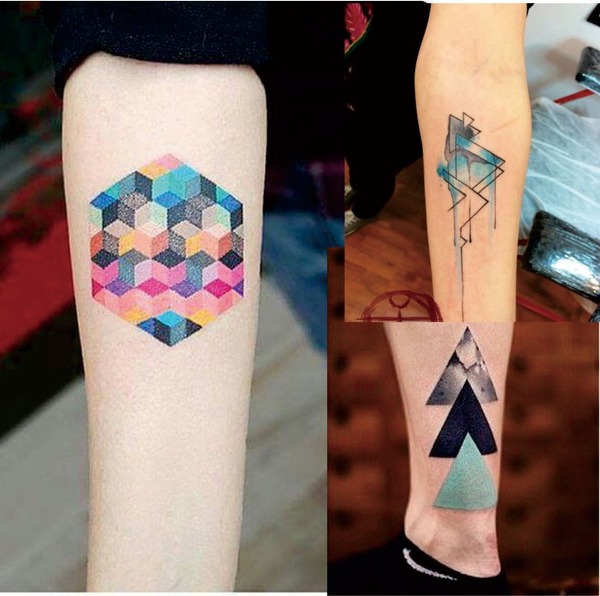This image showcases three different photos of geometric tattoos on a person with pale skin. On the left, there's a large vertical photo of a forearm featuring a colorful, 3D hexagonal design. The hexagon is composed of intricate, cube-like patterns in shades of teal, blue, pink, and purple, creating a striking, modern look. To the right of this image, there are two smaller photos stacked vertically. The top photo displays another forearm tattoo with minimalistic triangle designs, including a solid gray triangle and a blue triangle with a dripping effect, presenting a sleek, contemporary style. The bottom photo shows an ankle adorned with a tattoo of three stacked triangles, each with distinct patterns and colors—stone, black, and teal. The presence of a Nike sock confirms that this photo is of a leg. Together, these images highlight the person's collection of vibrant and geometric-themed tattoos.